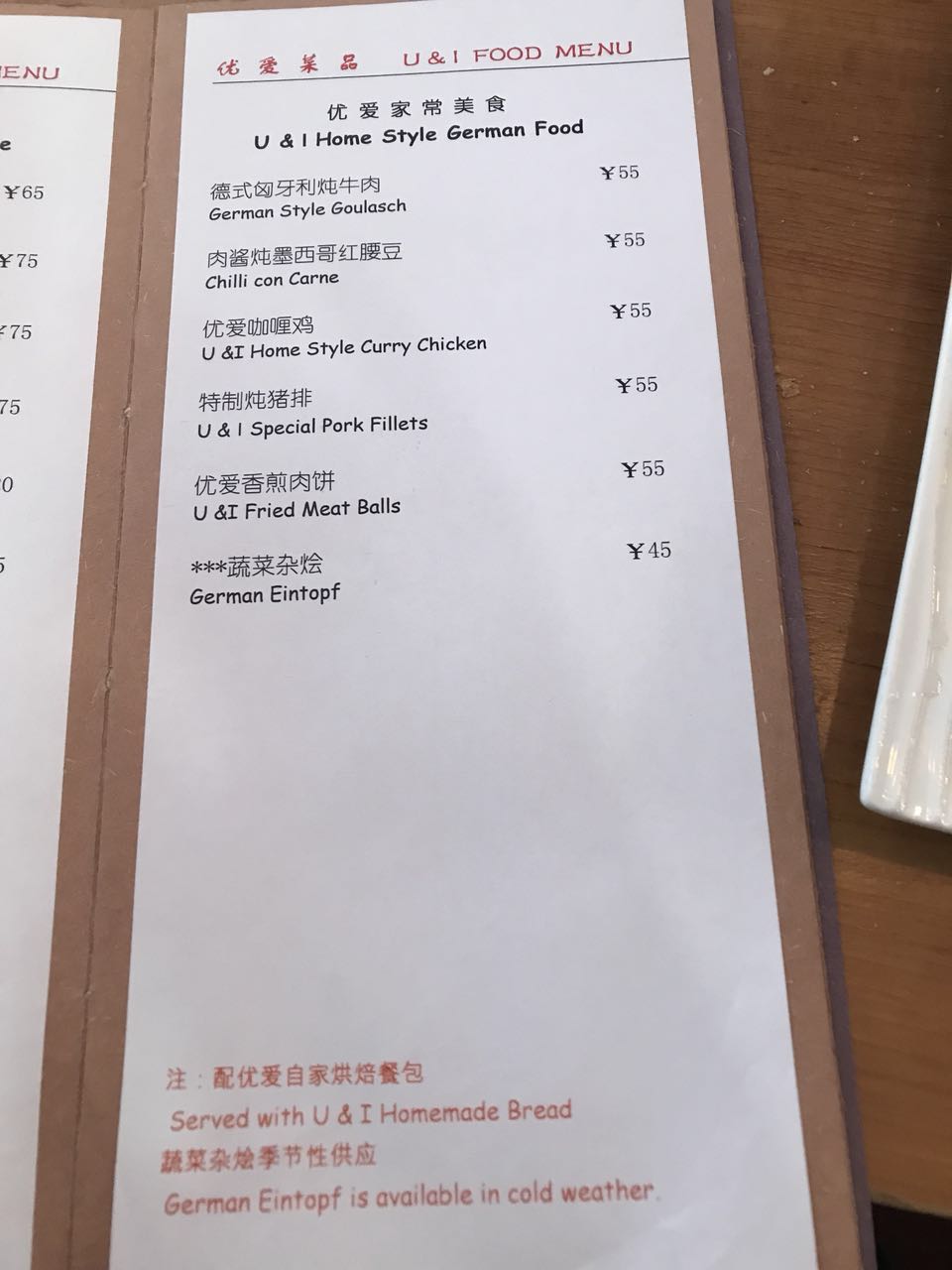This image depicts a menu for a restaurant specializing in homestyle German cuisine, with a touch of Chinese influence. The topmost section of the menu features Chinese characters, followed by the English words "You & I Food Menu." Below this header, additional Chinese characters translate to "You and I Homestyle German Food."

The menu offers six specially curated dishes, each listed in both its original language (possibly German) and its English translation:

1. **German-style Goulash** - 55¥ 
2. **Chili Con Carne** - 55¥
3. **You & I Homestyle Curry Chicken** - 55¥
4. **You & I Special Pork Fillets** - 55¥
5. **You & I Fried Meatballs** - 55¥
6. **German Eintopf** - 45¥

Each dish is priced with a currency symbol resembling a 'Y,' indicating it may be priced in Yen. 

At the bottom of the menu, there are more Chinese characters with the English translation indicating that all dishes are "Served with You & I Homemade Bread." Additionally, it notes that the "German Eintopf is available in cold weather."

The menu itself is designed to be tall and narrow, printed on white paper with black text, and is set against a brown background, giving it a simple yet elegant presentation.